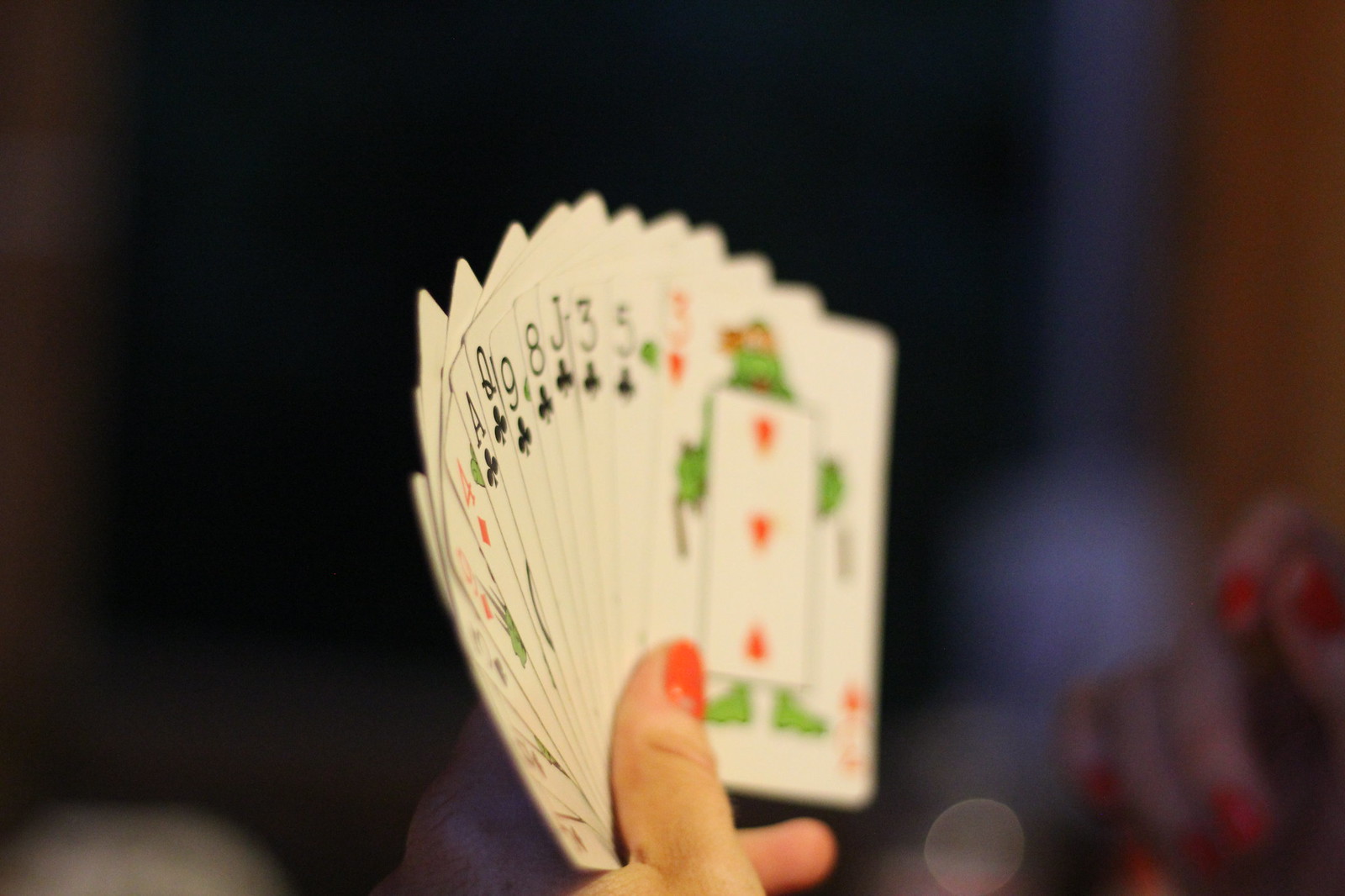In this evocative photograph set against a stark black background, a hand adorned with striking bright red nail polish holds a splayed fan of classic playing cards. The surrounding ambiance is shrouded in darkness, punctuated by an ethereal blue line and a dimly lit, warm wooden streak faintly visible in the backdrop. A soft, diffused blob of light illuminates the bottom left corner, subtly contrasting the hand's vivid hue on the extreme right edge. The playing cards, crisp and white, showcase a variety of faces with legibly displayed values: the Four of Diamonds, Ace of Clubs, Queen of Clubs, Nine of Clubs, Eight of Clubs, Jack of Clubs, Three of Clubs, Five of Clubs, and Three of Hearts. The overall composition hints at a moment of intrigue, perhaps mid-game, emphasizing the classic allure and mystique of card playing.